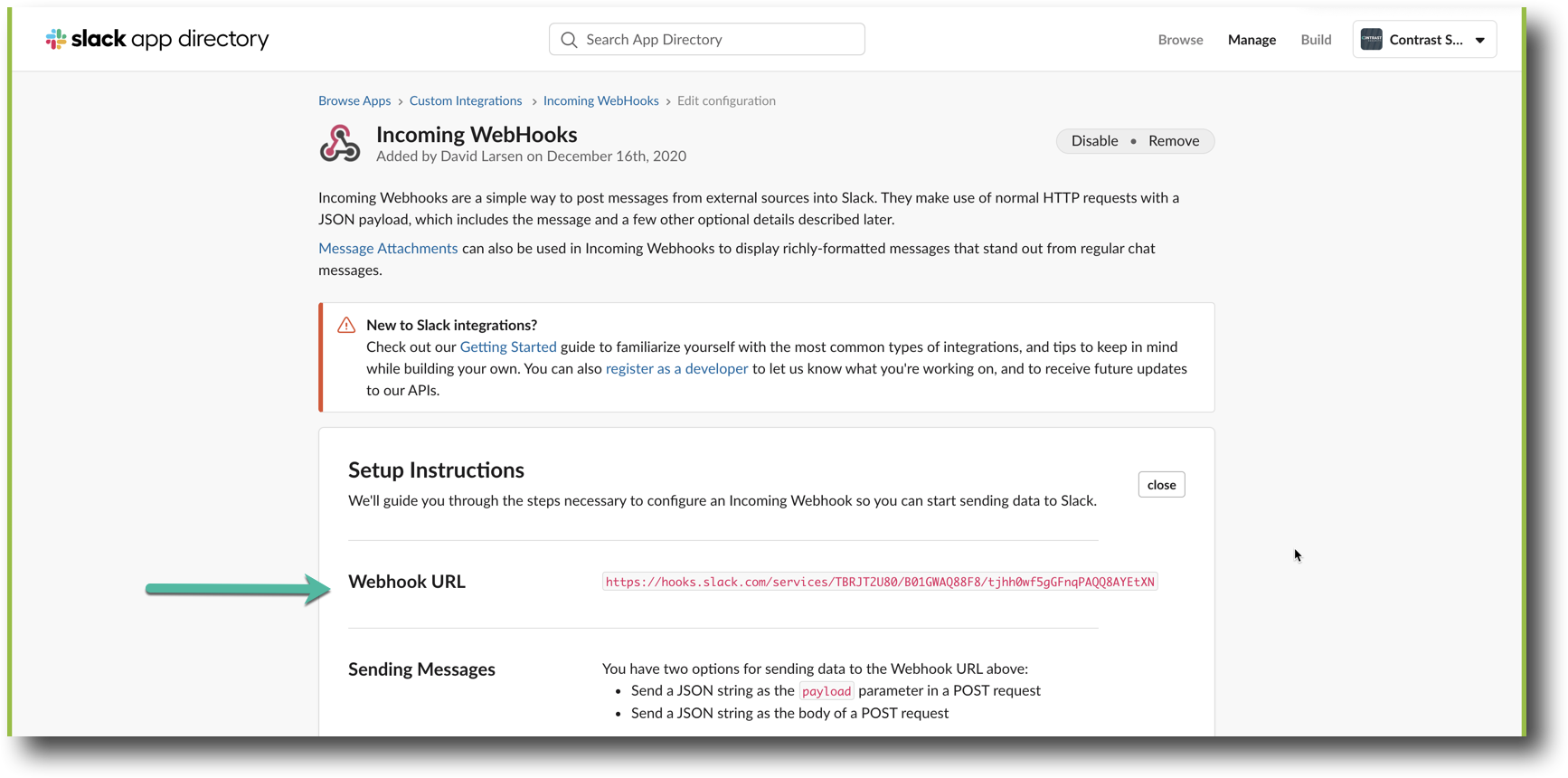The top section of the interface features a white background. In the upper left corner, "Slack" is prominently displayed in bold black text. Adjacent to it, "App Directory" is written in regular black text. To the right, there's a white search bar with a gray border and a gray magnifying glass icon, labeled "Search App Directory."

Below this, the header includes three tabs: "Browsing" in gray, "Managing" in black, and "Building" in gray, separated by a thin gray line spanning the width of the section. The background color shifts to gray after this point.

Centrally located, there is a blue banner with options such as "Browse Apps," "Custom Integration," and "Incoming Webhooks." Additionally, "Edit Configuration" is written in gray.

Underneath this banner, the title "Incoming Webhooks" is displayed in black, followed by the text "Added by David Larson, December 16, 2020." A descriptive paragraph explains, "Incoming webhooks are a simple way to post messages from external sources into Slack. They utilize standard HTTP requests containing a JSON payload, which includes the message and other optional details." The text "message attachments" appears in blue, followed by additional information in black, noting that these attachments can be used with incoming webhooks to deliver richly formatted messages, making them distinct from regular chat messages.

Towards the bottom, there's a section that guides new users with the statement, "New to Slack integrations? Check out our Getting Started guide to familiarize yourself with the most common types of integrations and useful tips for creating your own."

Finally, there is a "Setup Instructions" area at the bottom, which promises to guide users through the necessary steps to configure incoming webhooks, enabling them to start sending data to Slack seamlessly.